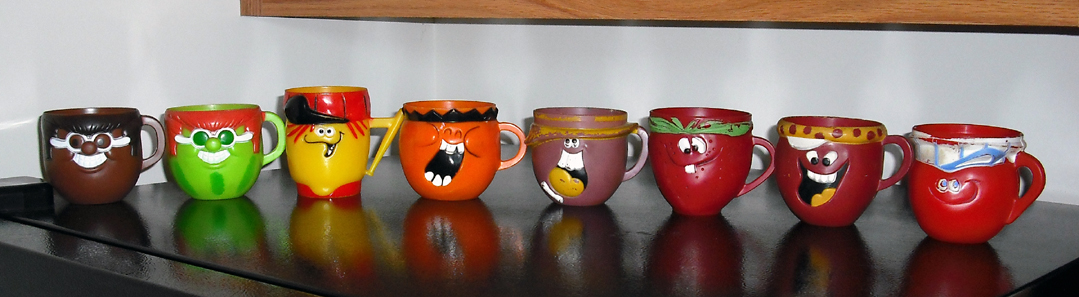This image features a row of eight novelty coffee mugs, each uniquely colored and adorned with a distinct, humorous face depicting a variety of expressions. Starting from the left, the first mug is brown with black hair, large white teeth, and brown eyes. It wears white glasses, highlighting a broad smile. The second mug is green, sporting red hair, glasses, and a comical expression with prominent teeth and a visible nose. The third mug is a combination of orange and yellow, characterized by a quirky face with small eyes and a peculiar smile beneath a red cap. The fourth in line is purely orange with an exaggeratedly open mouth, showcasing its cheeks in a playful manner. Next is a purple mug munching on a cookie, adding to the ensemble's whimsical charm. This is followed by a strawberry-themed mug that appears dizzy, featuring a single tooth protruding from its otherwise closed mouth. The burgundy mug has minimalistic features with small eyes and an open mouth revealing its tongue; the top is adorned with yellow and red dots. Finally, the lineup concludes with a bright red mug topped with white, whose gentle smile completes the array of lively expressions. All mugs have handles and their reflections can be seen on the shiny black surface they rest on.